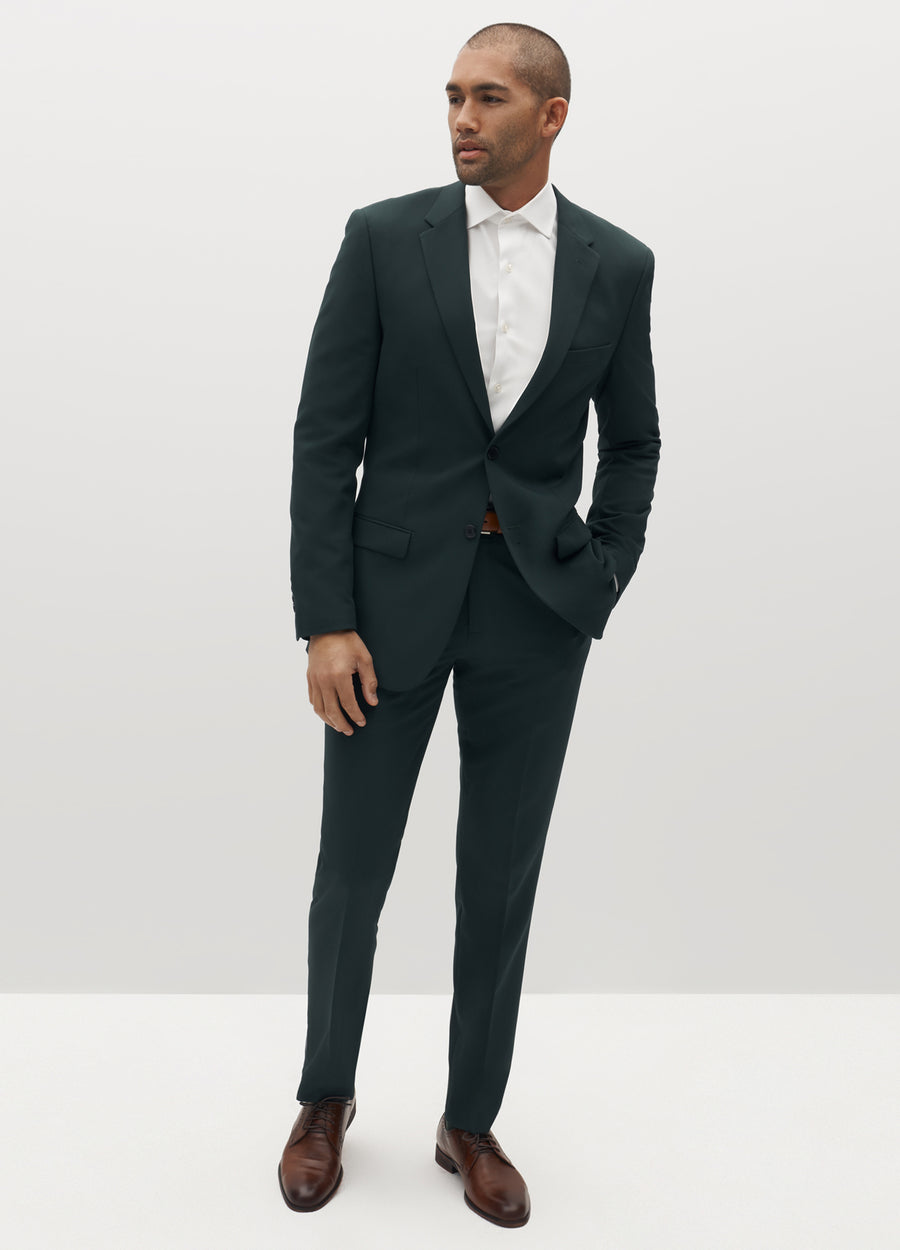The image depicts a man with tan, medium-dark skin standing against an all-white backdrop. He is dressed in a sharply tailored black suit, consisting of a jacket and matching pants, along with a white button-up collared shirt underneath. He wears a brown belt and shiny brown dress shoes that complete his ensemble. His hair is closely cropped in a buzz cut, and he has a short stubble covering his face, resembling a five o'clock shadow. The man is posing in a modeling stance, with one hand placed in his pocket causing the jacket to bunch up slightly, and the other hand resting by his side. He gazes off to his left, contributing to a polished and thoughtful demeanor. This elegant and poised appearance is reminiscent of an advertisement for high-end men's fashion retailers.